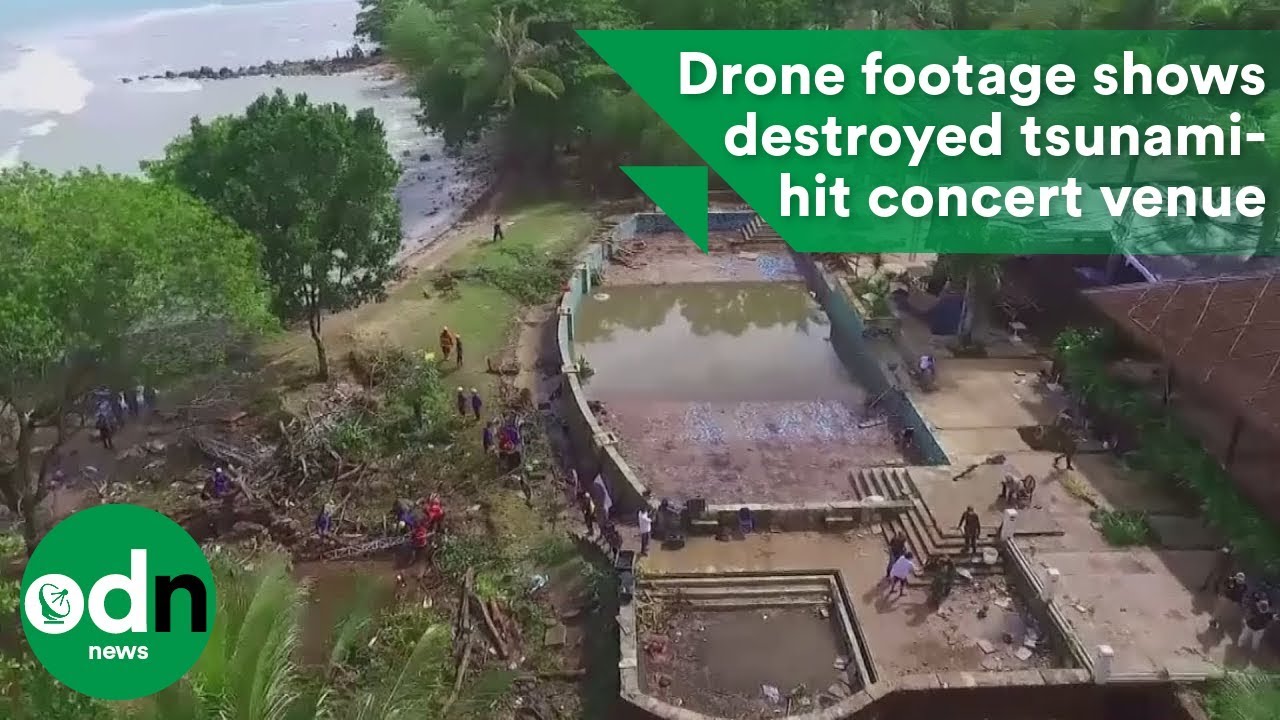The overhead drone footage captures the devastating aftermath of a tsunami-hit outdoor concert venue in Japan. The image showcased in the news clip, tagged with "O-D-N News" in white letters inside a green circle, alongside the logo, emphasizes the phrase, "drone footage shows destroyed tsunami hit concert venue" at the top right. The scene portrays extensive flood damage with the concert area submerged under dark, sandy seawater. Surrounding the venue, numerous palm trees lie destroyed, and green fields give way to brown-trunked trees, while a dark body of water looms on the right. To the left, the endless ocean, marked by a small sandy beach, stretches into the horizon, a stark reminder of the tsunami's origin. People scattered in and around the venue assess the catastrophic damage amidst the widespread devastation.